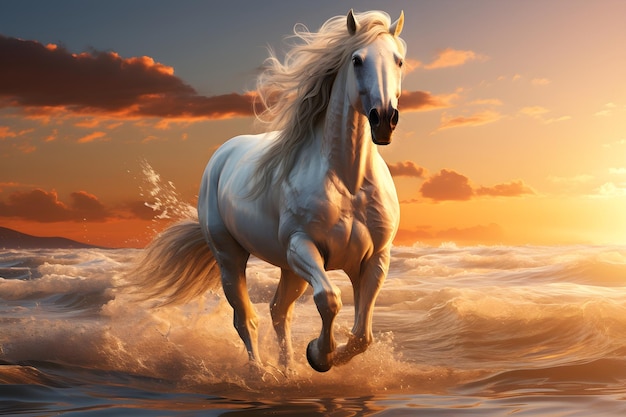This vibrant, computer-generated illustration depicts a powerful, muscular white stallion with a flowing, grayish-white mane and blond tail, mid-stride as it gallops through shallow waters near a beach. The horse features subtle black markings around its nose and mouth, while its muscular build is highlighted by bulging muscles and visible veins. The crashing waves splash around the horse's hooves and tail, emphasizing its dynamic movement. The horse's raised front hooves suggest a moment caught in mid-trot, with its head slightly turned to the right. The background showcases a breathtaking sunset sky infused with hues of orange, purple, blue, and cream. The sun, positioned just above the horizon, casts a warm glow, accentuating the clouds with orange highlights. To the left of the scene, a hill rises from the water, adding to the dramatic coastal setting. In the distance, the silhouette of a mountain further enhances the picturesque landscape.